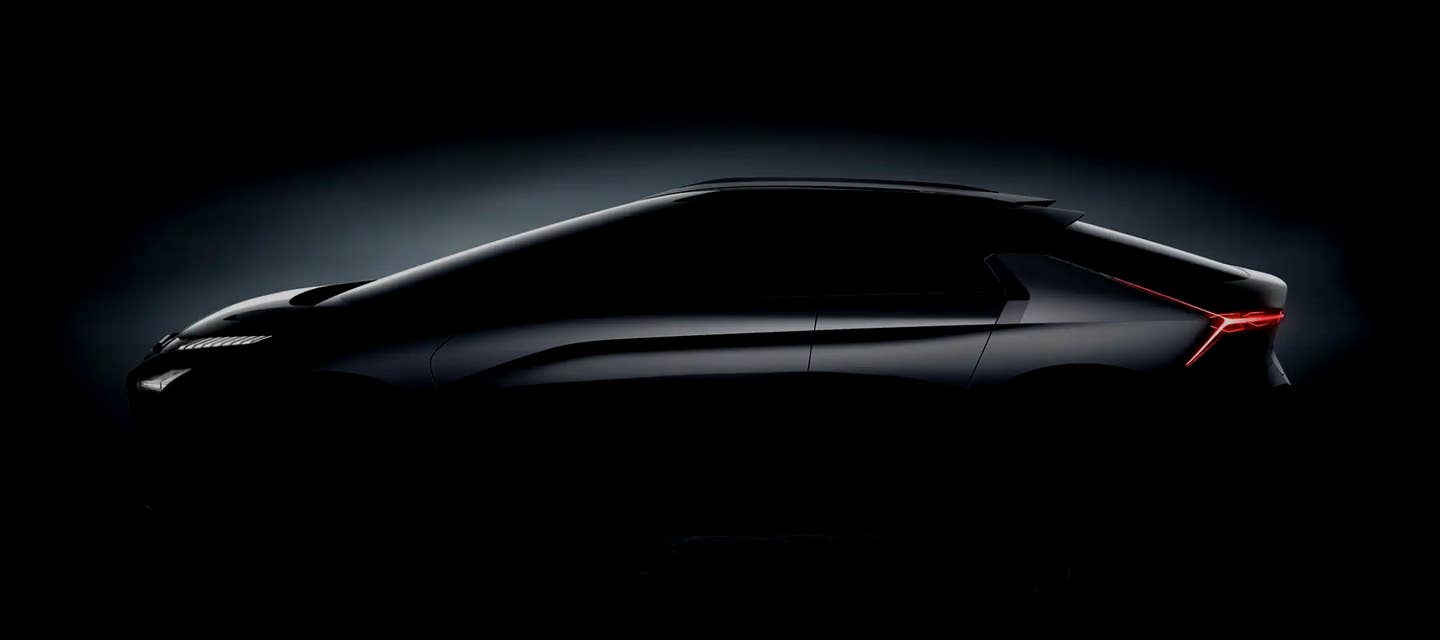The image features a sleek, black car set against a completely black background, almost creating a silhouette effect. The car, reminiscent of Batman's, exudes a stealthy, futuristic vibe. The body of the vehicle is modernistic and smooth, designed for a high-speed, almost invisible drive. The windows are entirely blacked out, preventing any view inside, and adding to its enigmatic appearance. Hints of light break through the darkness, with sharp white headlights illuminating the front and glowing red taillights at the back, suggesting the car is powered on. The car is viewed from the side, facing left, and the dark surroundings obscure the tires, making them blend seamlessly into the blackness. A subtle reflection of light off the car's surface barely separates it from the night, creating a ghostly yet striking visual.